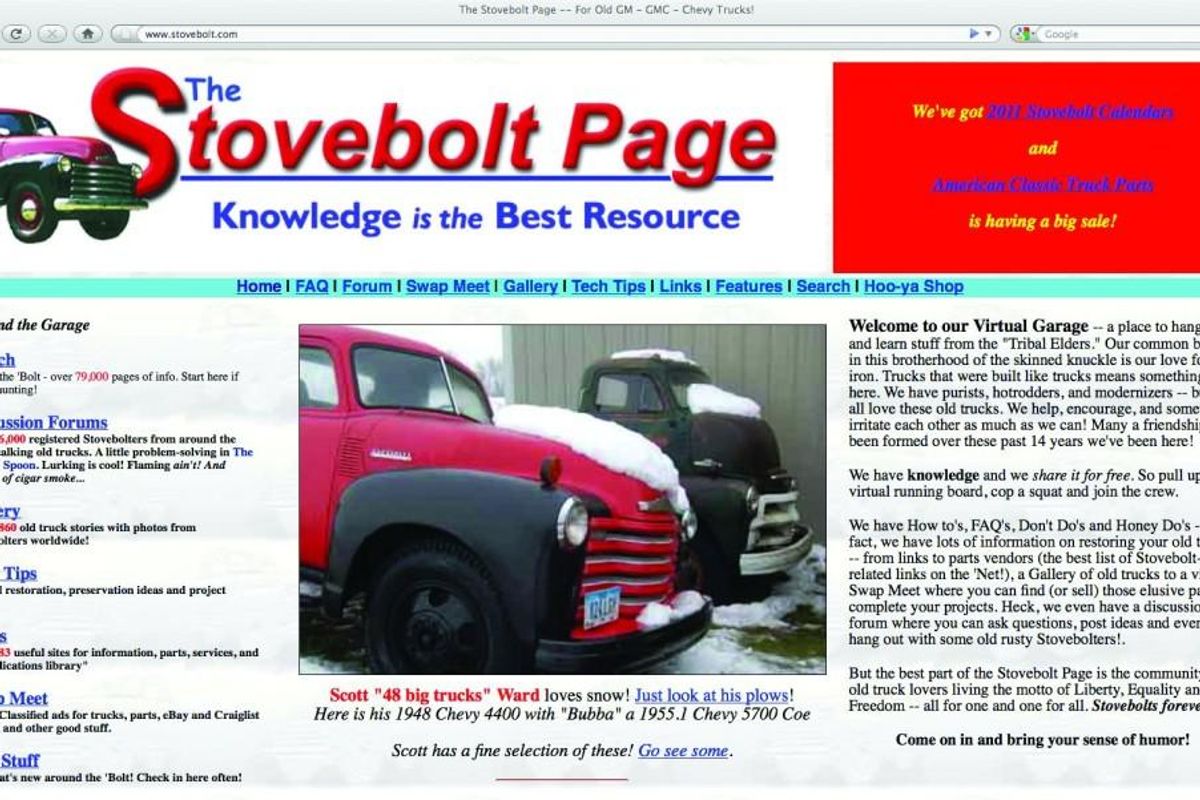This image is a screenshot of a webpage displayed on a Macintosh computer, distinguished by the characteristic grey Macintosh search bar at the top, with a Google search bar integrated on the far right. The webpage, titled "The Stovebolt Page -- For Old GM--GMC--Chevy Trucks!" is accessed via www.stovebolt.com and celebrates classic trucks. It showcases a white background with logos at the top corners: the upper left features a stylized image of a vintage black, red, and silver GM or Chevy truck, while the upper right contains an advertisement in a red rectangle, boasting in gold and black fonts about the 2022 Steve Bolt calendars and a big sale on American classic truck parts.

Below the header is a blue navigation bar, offering buttons for Home, FAQ, Forum, Swap Meet, Gallery, Tech Tips, Links, Features, Search, and Shop. The center of the webpage features a photo of two vintage trucks. The first truck, partially cut off by the picture’s framing, has a red grille, hood, and body with black fenders, wheels, and front bumper. The second truck, also only partly visible, is black and green with a gray grille, bumper, black fenders, and hood. Both trucks are parked by a gray corrugated metal building and are dusted with snow.

Further on the page, under the header "Welcome to our virtual garage," the text invites enthusiasts to join the community focused on the restoration, preservation, and enjoyment of classic trucks. This section mentions available resources, including how-to guides, FAQs, and links to parts vendors. The community celebrates a shared passion for old trucks, encouraging members to participate in forums, share projects, and engage in discussions, embodying the spirit of camaraderie and shared knowledge.